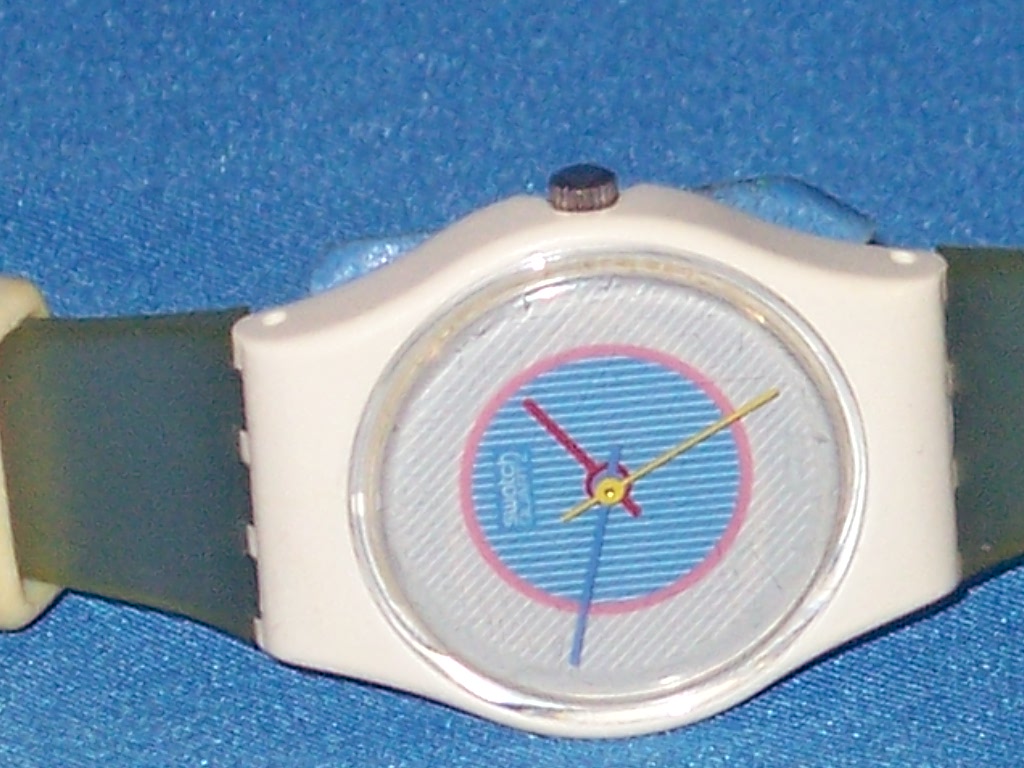This close-up photograph captures an exquisite wristwatch resting on a textured blue fabric surface. The high-level zoom reveals the intricate weave of the blue and white textiles beneath the watch. Positioned on its side, the watch's dark gray straps extend horizontally to the left and right of the frame. The watch face features a clear, protective covering that reveals a multi-colored center design, dominated by shades of gray, blue, and white, with various concentric circles adding depth. The watch's hands are vividly colored in red, yellow, and blue, standing out against the muted background. A small silver dial adds a touch of elegance to the white center area, completing the sophisticated look of the timepiece.